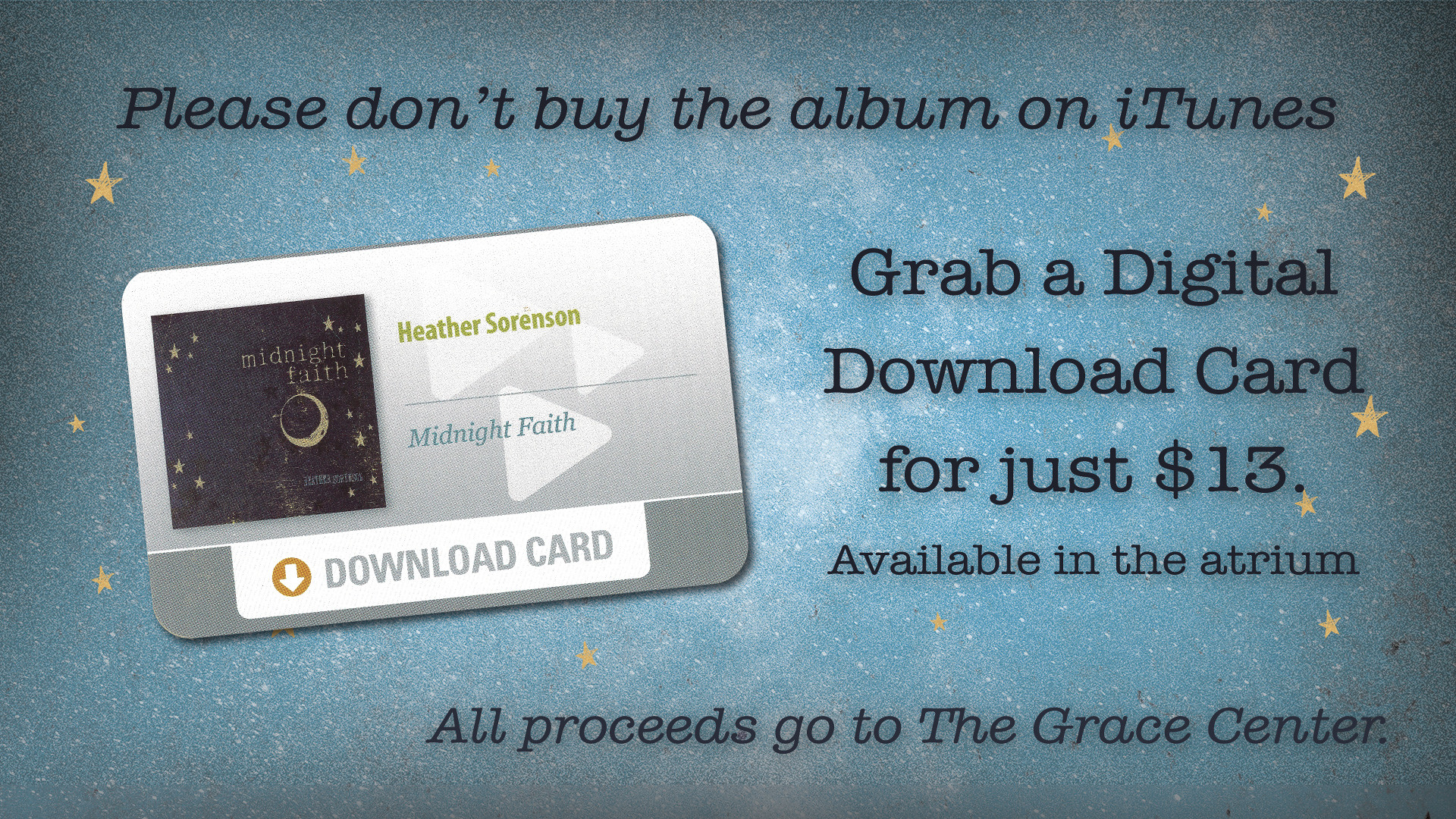This digital advertisement is a wide rectangular image featuring a textured light blue background speckled with white and adorned with small, five-pointed gold stars scattered throughout. At the top, in a curly black font, it reads: "Please don't buy the album on iTunes." Below this message, the text continues, "Grab a digital download card for just $13. Available in the atrium. All proceeds go to the Grace Center," also in black lettering.

On the left side of the image is a slightly tilted, gray card-shaped drawing. The top left of the card features a black square with small gold stars and the text "Midnight Faith" in gold font. Beside this square, in goldish or greenish letters, are the words "Heather Sorensen," indicating the artist. The card's bottom section also displays the words "download card" in gray, with an orange or yellowish circular arrow pointing left.

The card prominently showcases the album cover within the black square, depicting a moon in silhouette during a lunar eclipse, surrounded by gold stars. Overall, this visually rich advertisement encourages viewers to purchase the digital download card, with all proceeds supporting the Grace Center.